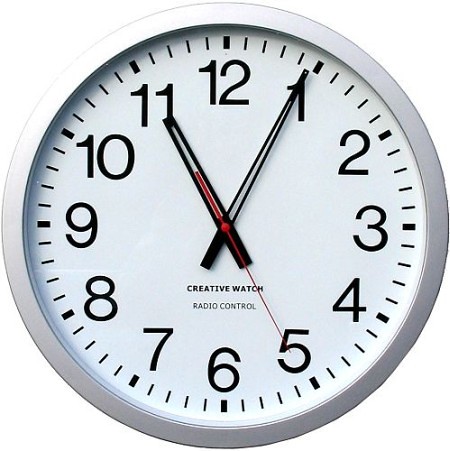This image showcases a contemporary clock illuminated by light from the left side. The clock's casing, which has a shiny finish making it difficult to discern whether it is white or silver, surrounds a pristine white clock face. The clock hands exude a futuristic aesthetic with their black outlines and white centers. Notably, the second hand features a striking design with its lower half colored red, extending down to a red central pivot. The minute hand is positioned just past the 5-minute mark, indicating that the time is approximately 11:04. The clock's bold, easily readable numbers enhance its clear design. The phrase "Creative Watch Radio Control" is inscribed on the clock face, signifying that it is a radio-controlled timepiece that automatically maintains accurate time.